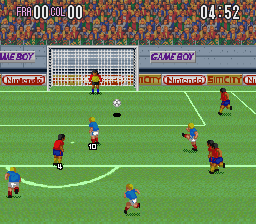This is a detailed still image from a Nintendo Game Boy soccer game. In the foreground, a vibrant green soccer field is depicted, adorned with precise white lines that demarcate various areas of play. On the field, multiple players are actively engaged in the game, sporting distinct uniforms: some wear red tops paired with blue shorts and black shoes, while others are clad in blue tops with white shorts and red and black shoes. 

In the background, a diverse crowd of spectators fills the stands, adding to the lively atmosphere. The upper left corner of the image displays the score "FRA00COL00" in white text, while the upper right corner shows a game time of "04..52". Additionally, advertisements for "Game Boy" and "Nintendo SimCity" can be seen in the background, enhancing the nostalgic feel of the scene.